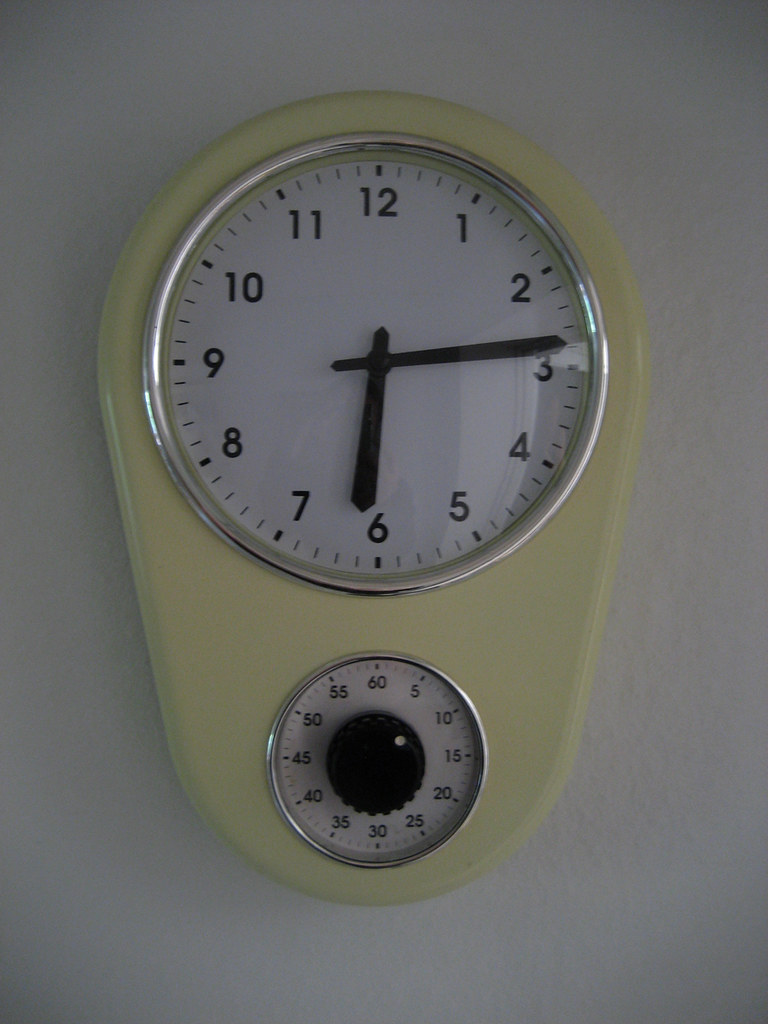This photograph features a decorative wall clock with a vibrant yellow outline. The main body of the clock is white and displays black numerals for easy readability. It is set within a yellow casing, adding a touch of brightness and style, making it suitable for a kitchen setting. Beneath the clock face, there is a second hand timer numbered from 5 to 60, which can be used for precise timing needs, such as cooking or baking. The clock displays the time as 6:14, though it is unclear whether it is in the morning or evening. The clock is mounted on a plain white wall, further accentuating its colorful design.